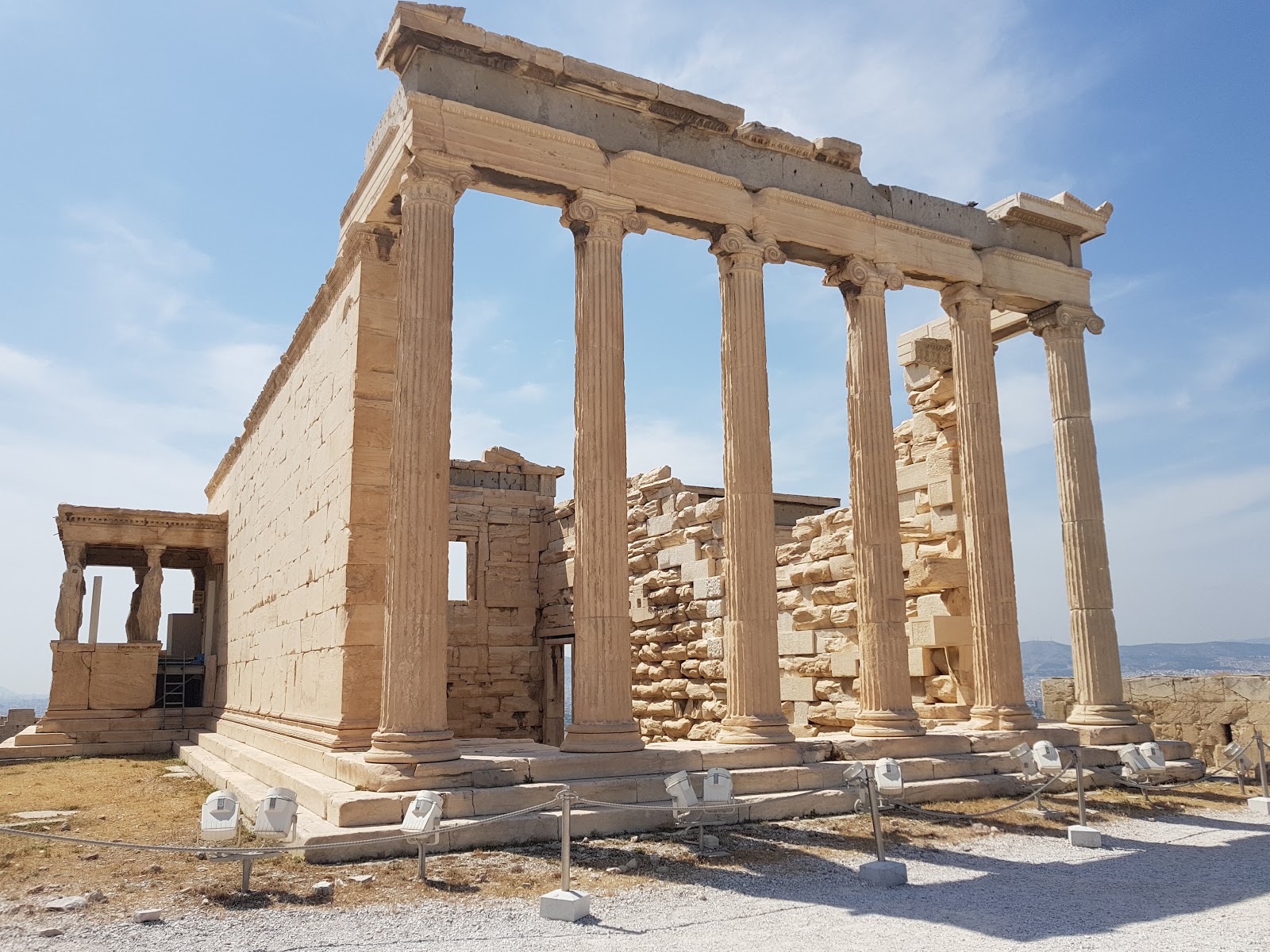The image depicts the front and side view of ancient ruins, possibly of a Greek temple, high up on a hill with mountains in the distance. The structure features six grand, cream-colored stone columns at the front, supporting archways, though the roof has long since collapsed. The main hall is large and open and extends to a smaller room in the back, where a single window is discernible. The left side of the temple has a smaller adjoining building, while another secondary exit is visible on the right. The structure lacks a complete wall due to partial collapse. The entrance to the temple is accessed via a flight of three steps. The area is roped off or fenced with a chain link barrier to prevent entry, hinting at preservation efforts. Spotlights illuminate the ruins, suggesting that evening tours might be available.